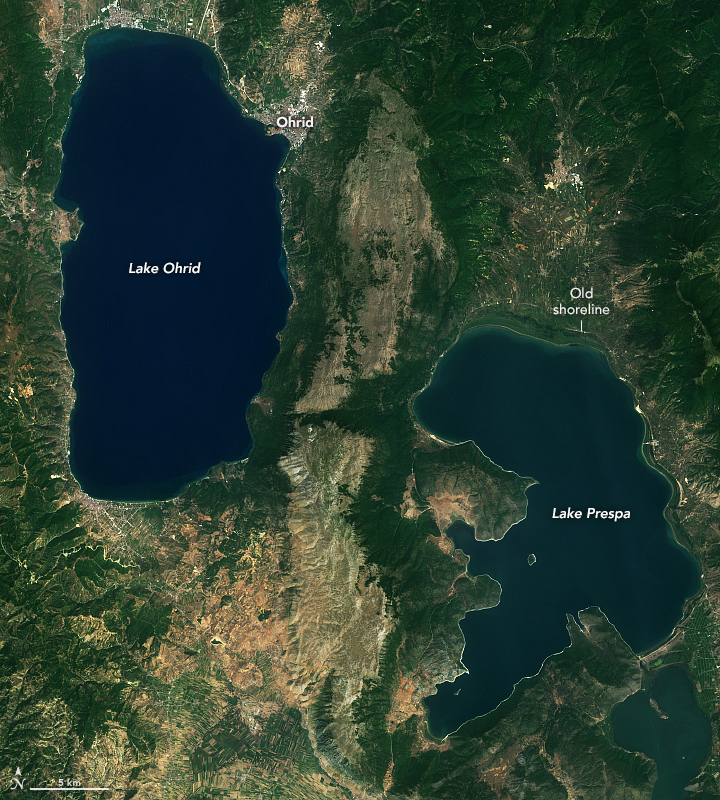This is an overhead satellite image showcasing two distinct lakes surrounded by a combination of landforms and vegetation. In the top left corner, the dark blue Lake Ohrid is prominently labeled in white letters, with the adjacent town of Ohrid also marked to the right of the lake. A larger, jagged-shaped lake named Lake Prespa is situated towards the bottom right, similarly labeled in white. Above Lake Prespa, the label "Old Shoreline" highlights a previous extent of the lake, indicating shrinkage over time. Separating the two lakes, mountain ranges with visible patches of exposed rock are evident, suggesting a rugged terrain. Surrounding these geographical features, vast expanses of green forests are interspersed with grasslands, particularly noted in the top and right-hand corners of the image. A watermark or logo is positioned in the bottom left of the photograph.